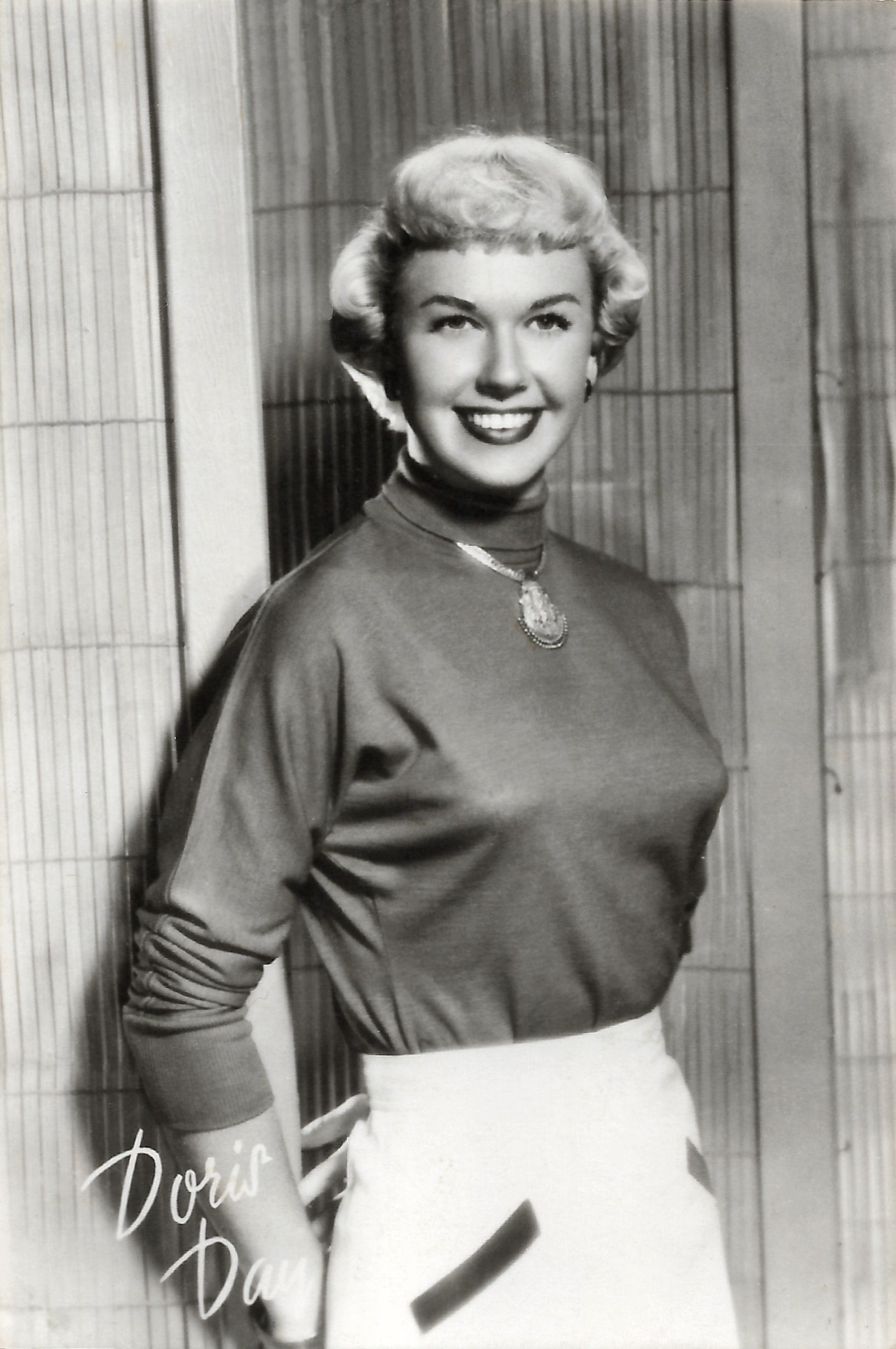The black-and-white photograph features the iconic actress Doris Day, renowned star from the 1950s and 60s. In this professionally taken, elegant promotional shot, Doris Day is posed gracefully, gazing slightly upward and smiling warmly, giving the image a genuine and inviting feel. Her blonde hair is styled in a classic, short coiffure with teased bangs and tight curls on either side, representative of the era’s glamorous aesthetic. She is dressed in a turtleneck sweater with its long sleeves casually rolled up to just below her elbows, paired with a light-colored skirt accented by dark pockets. Around her neck, she wears a pendant necklace that rests just below her collarbone, adding a touch of refinement to her ensemble. The backdrop appears to be a bamboo screen, which enhances the photograph's sophisticated yet casual vibe. An autograph by Doris Day is inscribed at the bottom left corner, further signifying the photo's promotional purpose. The photograph captures not only her timeless beauty but also her poised and charming demeanor, making it a treasured piece from the golden age of Hollywood.